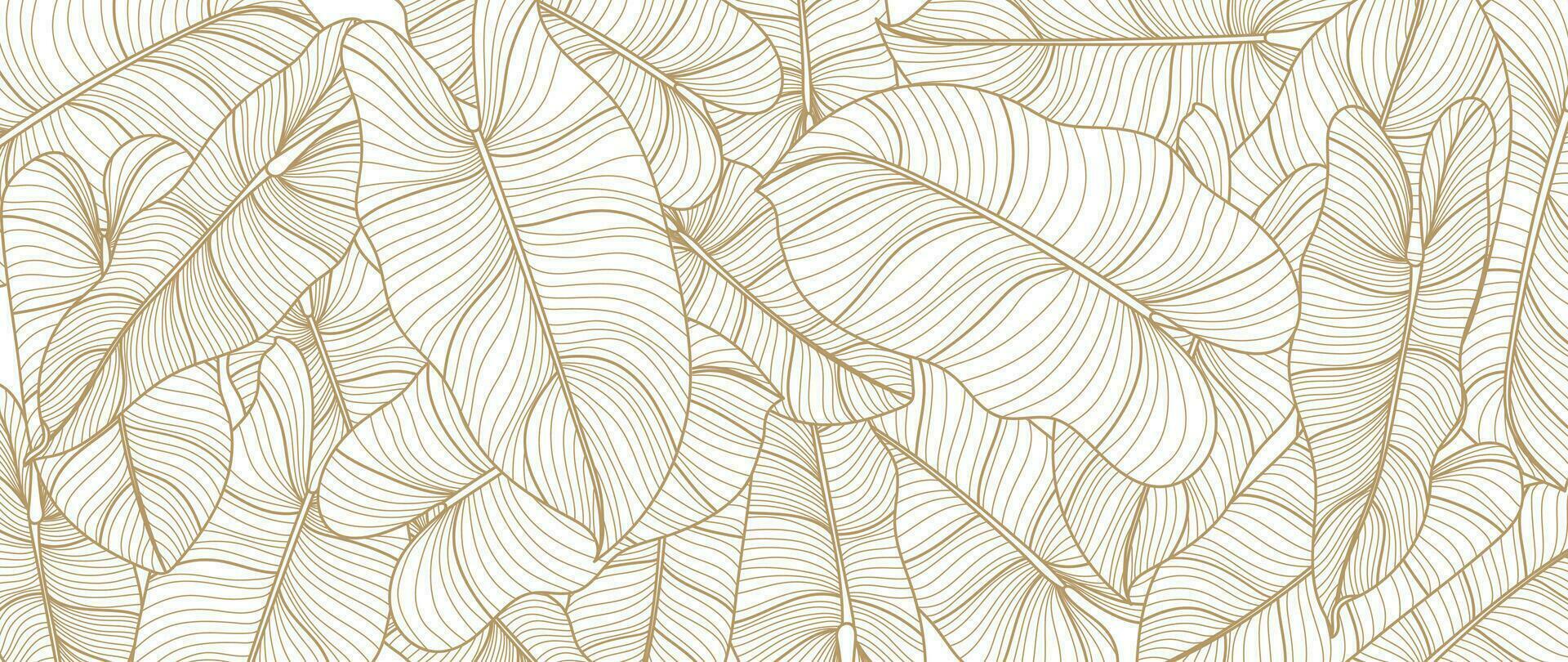The image is a highly detailed line drawing, possibly a digital or abstract design, featuring numerous palm fronds and elephant ear leaves. The leaves are primarily white with intricate gold outlines, highlighting the veins and edges. The composition is dense, with the leaves overlapping and covering almost the entire canvas, leaving very little negative space. The arrangement appears jumbled and unorganized, creating a layered, almost chaotic visual effect. Despite the complexity, there are a couple of prominent leaves, with one pointing down to the left and another to the right, standing out among the mass. The design lacks a filled background, emphasizing the line-drawn quality of the artwork. This could serve as a striking screensaver or wallpaper, given its detailed and abstract nature.